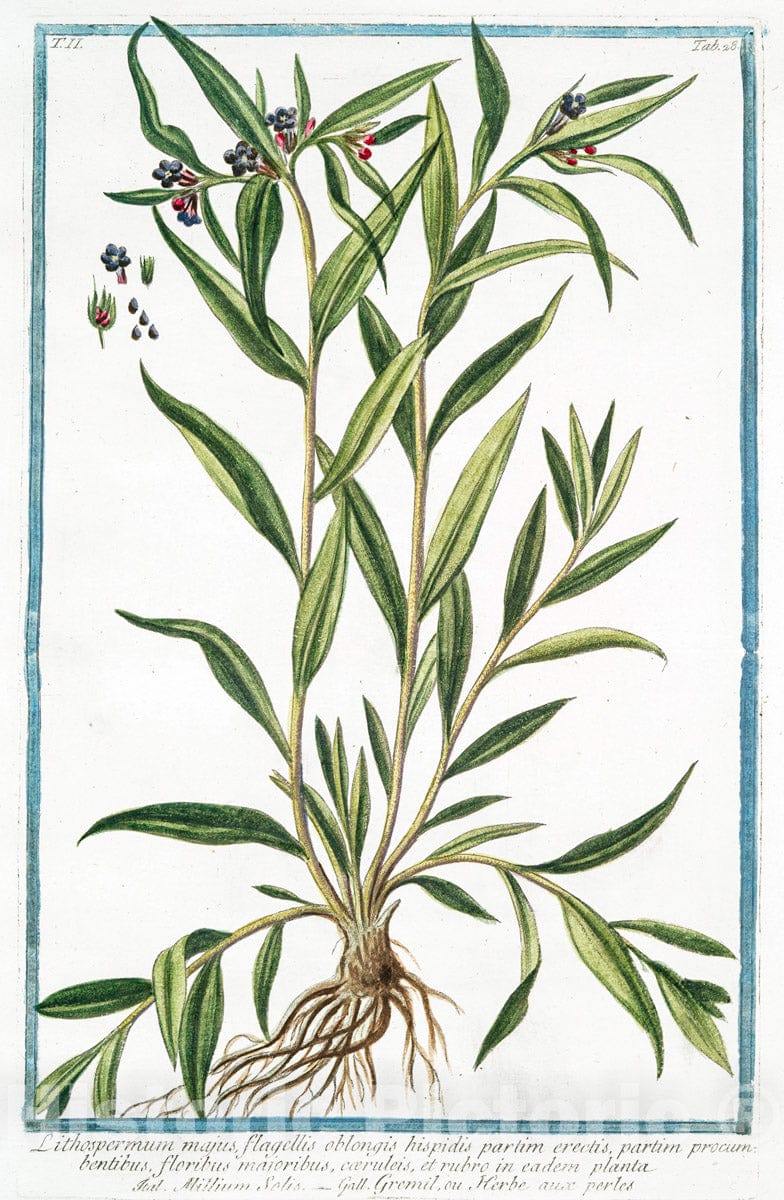This is a detailed botanical illustration on a white background, set within a medium blue border. The plant depicted has numerous stems of varying lengths, adorned with long, narrow green leaves. At the top of the plant, clusters of dark blue berries are visible, lending it a resemblance to bamboo, though the berries distinguish it from bamboo. There is a close-up view of these berries to the top left of the image, showcasing their detailed structure. The plant's root system is prominently displayed at the bottom, with a branching root ball. Underneath this, barely legible text in Latin is inscribed, suggesting a scientific annotation. The entire illustration is rendered in a vintage botanical style, emphasizing meticulous detail and subtle coloration, typically found in classical botanical prints.